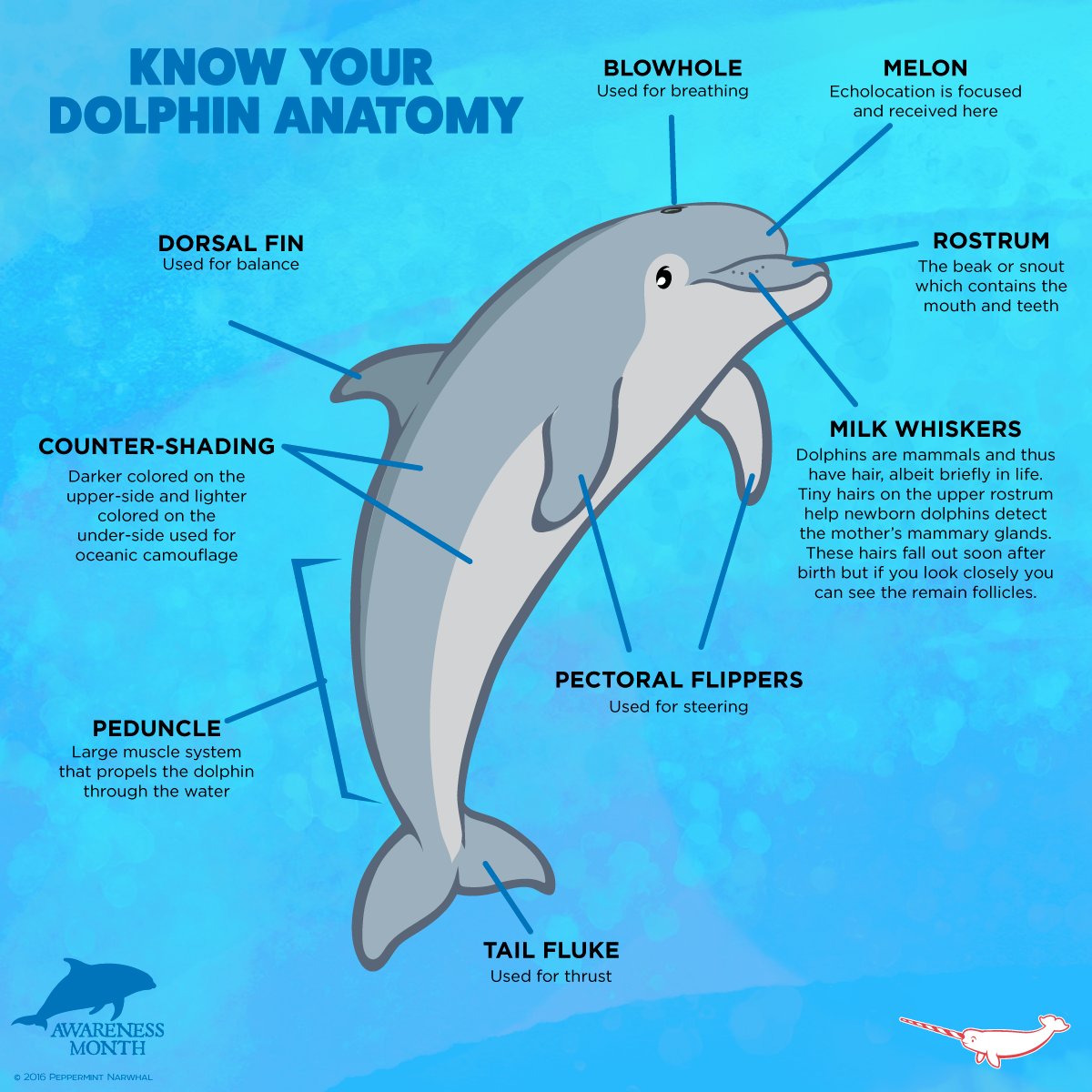This informational poster, set against a light blue splotchy background, is titled "Know Your Dolphin Anatomy" in the top left corner. It features a detailed illustration of a gray dolphin with various parts of its anatomy labeled in black letters. The diagram includes specific areas such as the Blowhole, used for breathing, and the Milk Whiskers. Labels also point to the Pectoral Flippers, Tail Fluke (used for thrust), the powerful Peduncle muscle system for propulsion, and the Dorsal Fin, critical for balance. Additional labeled features include the Melon, Rostrum, and Counter Shading. Each part is accompanied by a brief explanation of its function. At the bottom left, there is a small silhouette of a dolphin with the text "Awareness Month, 2016, Peppermint."